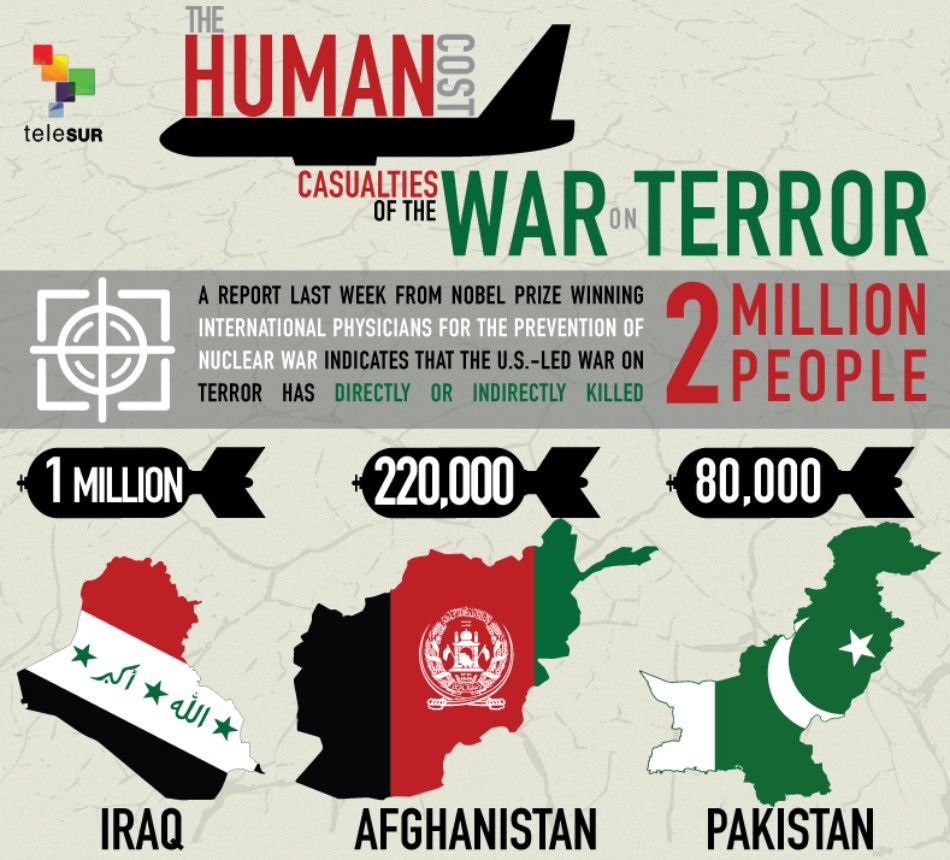The infographic titled "The Human Cost: Casualties of the War on Terror" features a visually compelling design centered around an alarming statistic. At the top, the title is arranged around the black silhouette of a military plane. In the upper left-hand corner, there's the logo of the organization TELASUR, comprised of overlapping squares in red, orange, green, purple, and light blue, with "TELA" in lowercase and "SUR" in uppercase. 

Beneath the title, a grayish banner spans the width of the graphic. On the left side of this banner, there is a white target symbol. The text within and around this banner, in varying colors—black, white, green, and red—states: "A report last week from Nobel Prize-winning International Physicians for the Prevention of Nuclear War indicates that the U.S.-led war on terror has directly or indirectly killed 2 million people," with "2 MILLION PEOPLE" standing out in large red letters.

Illustrations of stylized black bombs are positioned below this gray banner, each corresponding to different countries involved in the conflict. The first bomb on the left, marked with "1 Million" in white text, overlays a map of Iraq, represented with its flag featuring red, white, and green colors. The second bomb in the middle, marked "220,000" in white text, is overlaid on a map of Afghanistan, with its flag colored black, red, and green. The third bomb on the right, marked "80,000" in white text, overlaps a map of Pakistan, characterized by its green backdrop and white stripe and star. Beneath each map, the respective country's name—Iraq, Afghanistan, and Pakistan—is displayed in bold black letters.

The background of the entire infographic is a light greenish-gray, which offsets the multicolored elements, making the stark statistics stand out prominently.